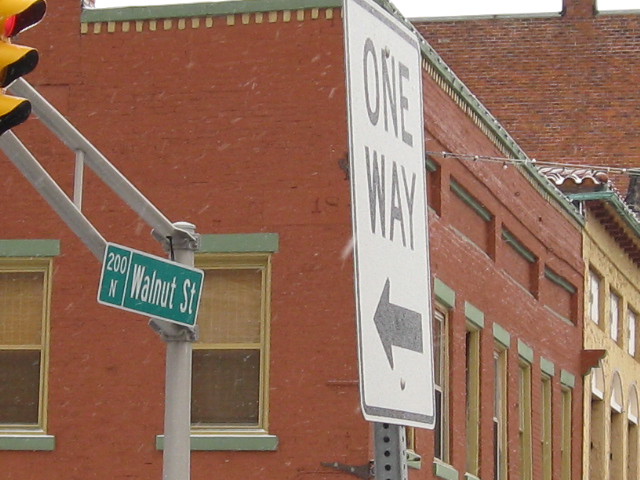The image captures the edge of a "One Way" street sign, which is oriented towards the camera and points to the left, indicating the direction of travel on Walnut Street. Positioned prominently in the foreground, the sign anchors a scene filled with urban details. Adjacent to the sign is a street lamp and a traffic light.

In the middle of the image, we see an older brick building with a flat roof and traditional windows, emblematic of a historic part of town. A street sign identifying the intersection as Walnut Street and 200 North is visible. Snow or sleet begins to fall, captured as fine, short diagonal lines against the red brick wall of the building.

In the right part of the image, festive Christmas lights or small string lights adorn the building, adding a touch of seasonal charm to the scene. In the background, another taller brick building looms, contributing to the overall impression of a quaint, older cityscape. Snowflakes create a magical atmosphere, transforming this urban moment into a picturesque winter setting on Walnut Street, 200 North.